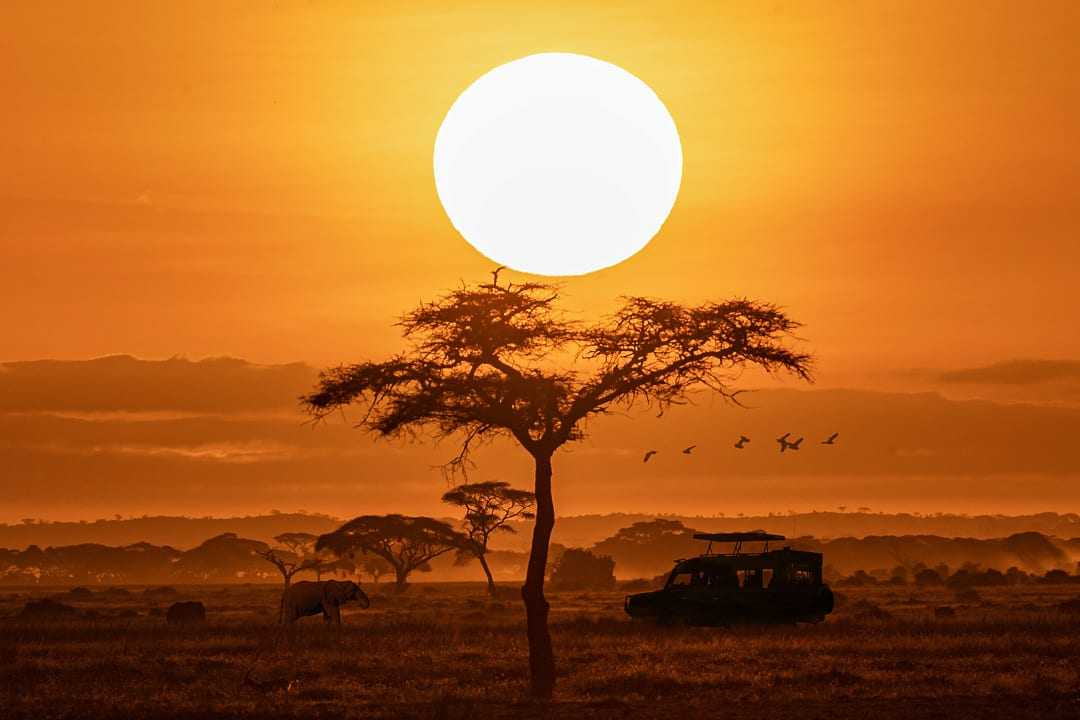The photograph captures a breathtaking sunset over the African plains, radiating a warm gradient from pure orange near the setting sun to a darker, more subdued orange towards the edges. Dominating the scene is a solitary, majestic tree silhouetted against the vibrant sky. To the left, an elephant stands prominently, while to the right, a vehicle, likely part of a safari expedition, casts the darkest shadow on the landscape. Silhouettes of birds fly above, adding to the tranquil and serene ambiance. The entire scene is bathed in a beautiful glowing orange hue, with the bright yellow sun at the center, creating a harmonious and peaceful tableau of nature.